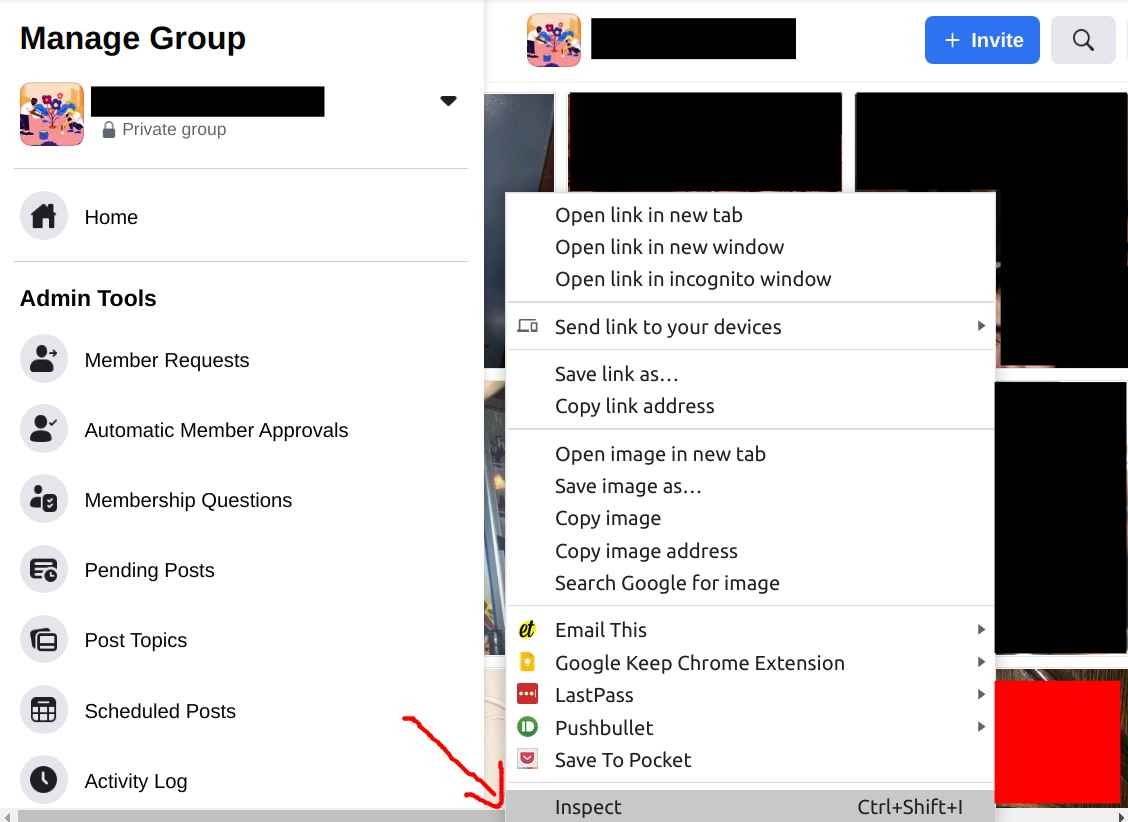Here is a precise and detailed caption for the described image:

---

The screenshot showcases the "Manage My Group" interface on a platform, indicating a private group setting. A diverse and inclusive icon of a group of people is prominently displayed, symbolizing collaboration within the group. The same icon is also positioned at the top center of the screen, partially obscured by a blacked-out bar. The interface provides an "Invite" function accompanied by a search bar. In the central pane of the screen, options for "Open Link in New Tab," "Open Link in New Window," and similar actions are listed. A red arrow points towards the "Inspect" option at the bottom of this list. On the left, under the "Home" section, several administrative tools are outlined, including "Member Requests," "Automatic Member Approvals," "Membership Questions," "Pending Posts," "Post-Atomic Topics," "Schedule Posts," and "Activity Log." Behind this, on the right side, a partially visible, additional tab with blanked-out pictures can be seen.